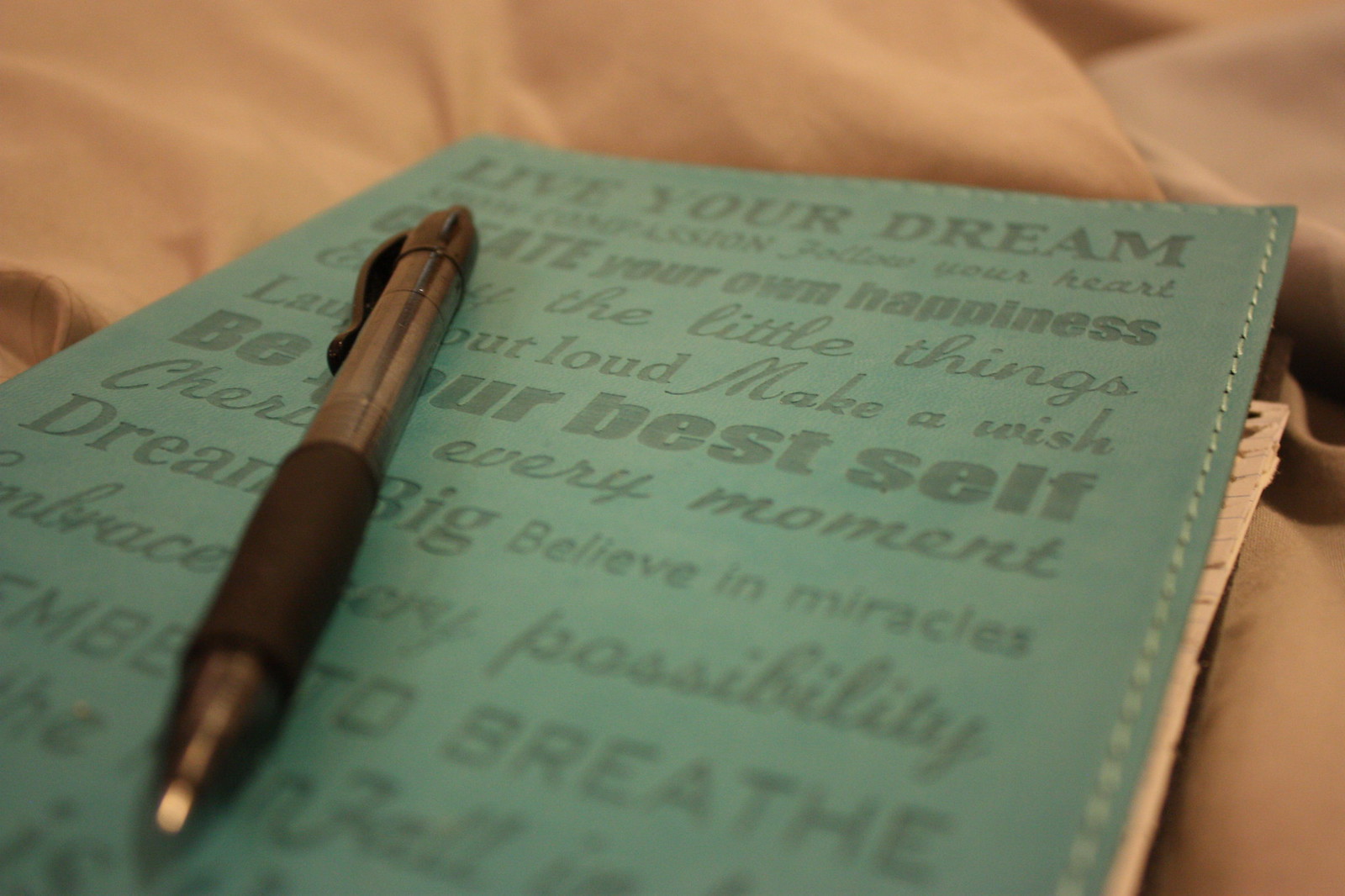This artistic photograph features a close-up of a worn, handmade journal with a leather cover adorned with positive sayings such as "live your dream, create your own happiness, be your best self, dream big, believe in miracles." The notebook, woven from bluish-green material with visible stitching along its top and right sides, suggests it's been well-used. A regular, slightly chunky black ballpoint pen with a rubber grip and clip rests diagonally on the journal's cover. The whole arrangement lies atop a light brown, possibly tan, fabric that appears to be a wrinkled and ruffled bedspread, adding to the intimate and cozy aesthetic of the scene. Pieces of paper peeking out from the journal further hint at its use as a personal space for thoughts and ideas.